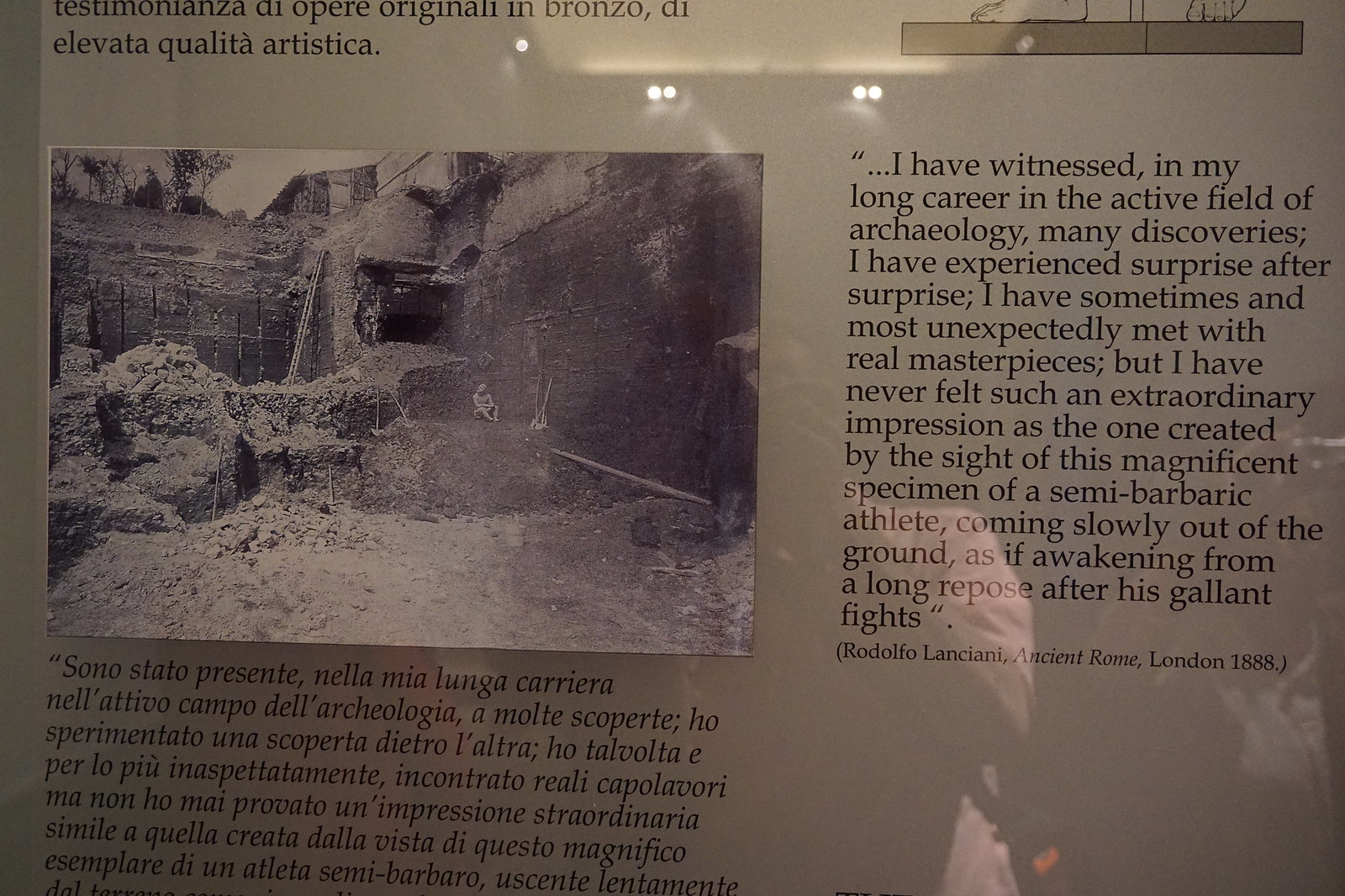The image showcases an informational plaque, likely photographed at a historic landmark, viewed on a computer screen with a noticeable glare. The plaque is set against a yellowed paper backdrop, resembling an old newspaper or magazine article. On the left side of the plaque, there is a prominent black and white photograph depicting an excavation site, possibly a mountainside with falling rocks and decaying buildings atop it. The site appears abandoned, revealing a person sitting on a dirt pile with a shovel, near a primitive wooden cabin. Below the photograph, there is an inscription in Italian, presumably a quote. To the right of this image, the English translation of the quote reads: "I have witnessed in my long career in the active field of archaeology many discoveries. I have experienced surprise after surprise. I have sometimes and most unexpectedly met with real masterpieces, but I have never felt such an extraordinary impression as the one created by the sight of this magnificent specimen of a semi-barbaric athlete coming slowly out of the ground, as if awakening from a long repose after his gallant fights." This quote is attributed to Rodolfo Lanziani, Ancient Rome, London, 1888. The detailed presentation and the excavation imagery suggest the plaque is part of a museum display intended to convey historical and archaeological significance.